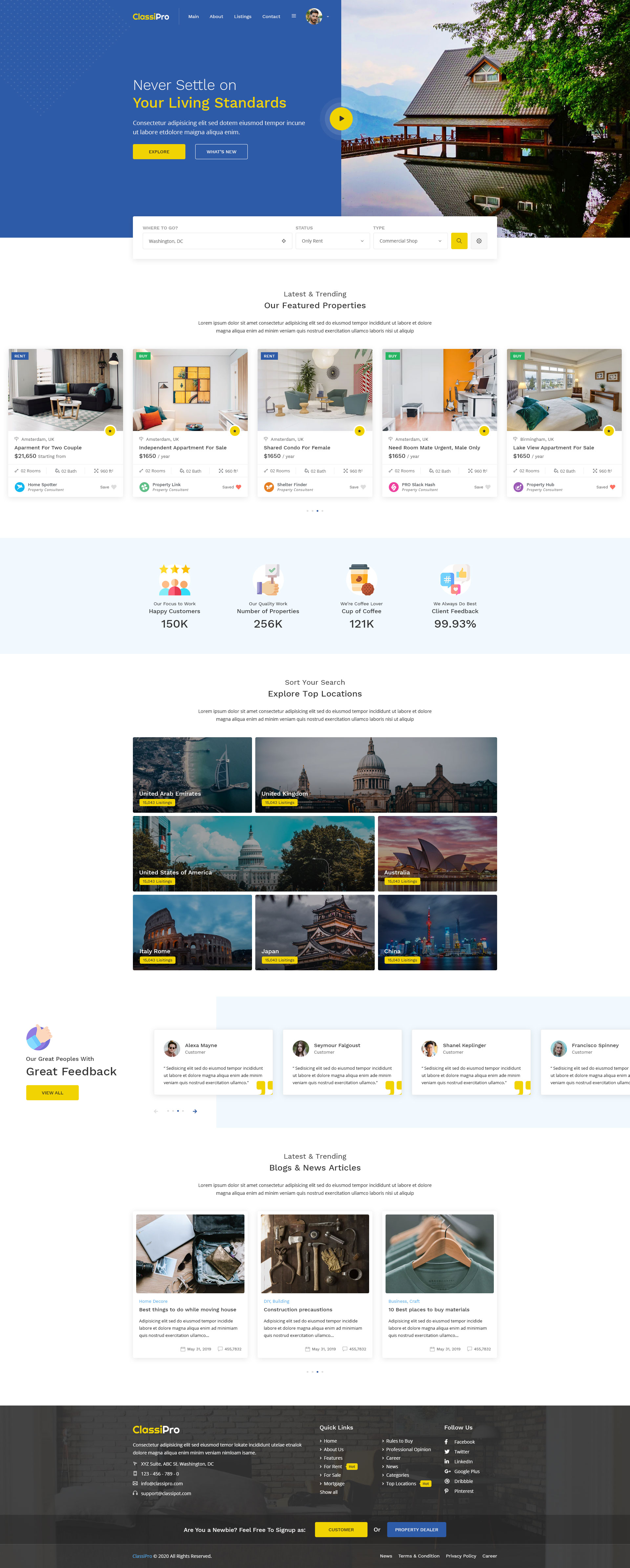The image is a vibrant, detailed color photograph of a website, likely captured from a cell phone, computer, or laptop screen. At the top, a rectangular banner on the right-hand side features a vivid image of a house. Adjacent to it, the left side of the banner has a solid blue background with the motivational text "Never settle on your living standards," accompanied by two checkboxes below.

Below the banner are five distinct screen captures showcasing different rooms, each accompanied by descriptions, costs, and presenter information. 

Beneath these room captures, there is a horizontal, light blue-filled rectangle displaying various statistics: 150K, 256K, 121K, and 99.93%, each with corresponding icons above them.

The next section features a mosaic of seven stunning photographs depicting iconic locations from around the world, including the U.S. Capitol, the Roman Colosseum, scenes from Japan, Australia, and more, each rendered in brilliant color.

Finally, the bottom of the image boasts the text "Great feedback," followed by four user surveys, illustrating the positive responses from different individuals.